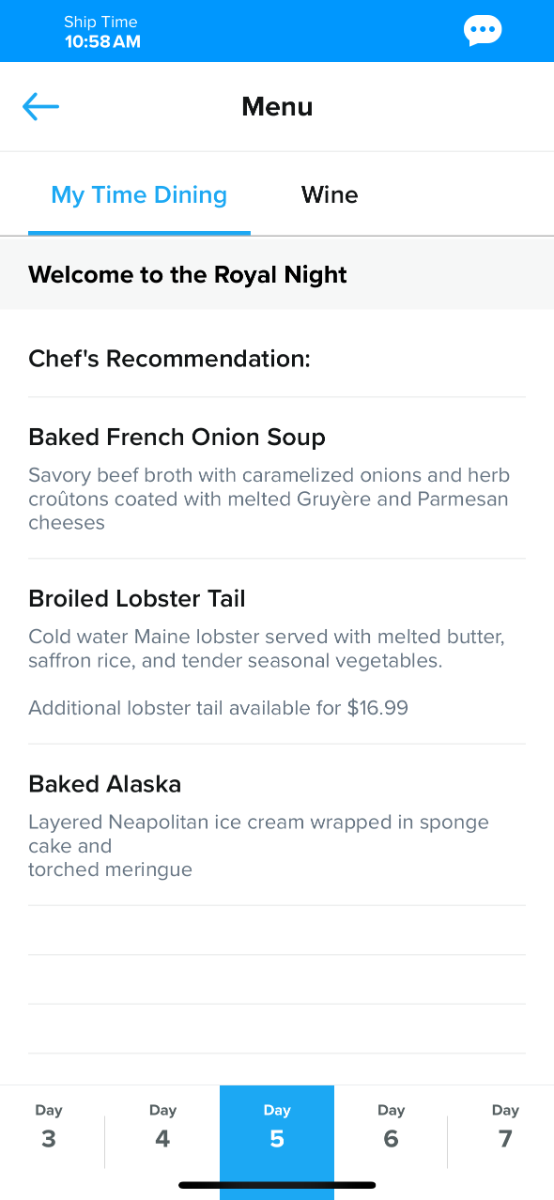Screenshot from a Mobile App

The screenshot shows a mobile app interface. At the top, there is a light blue border with text reading "Ship Time" and "10:58 AM." The time "10:58 AM" is displayed in a bold white font, distinguishing it from the lighter "Ship Time" text. In the upper right corner, a message icon is visible, featuring a white thought bubble with three blue dots inside, symbolizing unread messages or notifications.

Underneath the blue border, the interface transitions to a white background. At the top of this section, there is a blue back arrow next to the word "Menu" in black lettering. Below this, the text "My Time Dining" is prominently displayed in blue and underlined, followed by "and Wine."

The main content area welcomes the user with "Welcome to the Royal Knight" and lists the "Chef's Recommendations." The recommendations include:

- **Baked French Onion Soup:** A savory beef broth with caramelized onions and herb croutons, topped with melted Gruyere and Parmesan cheeses.
- **Broiled Lobster Tail:** Cold-water Maine lobster served with melted butter, saffron rice, and tender seasonal vegetables. An additional lobster tail is available for $16.99.
- **Baked Alaska:** A dessert featuring layered Neapolitan ice cream wrapped in sponge cake and covered with torched meringue.

At the bottom of the screen, it indicates "Day 5 of 34567" with "Day 5" highlighted in blue, marking the current day in the dining itinerary.